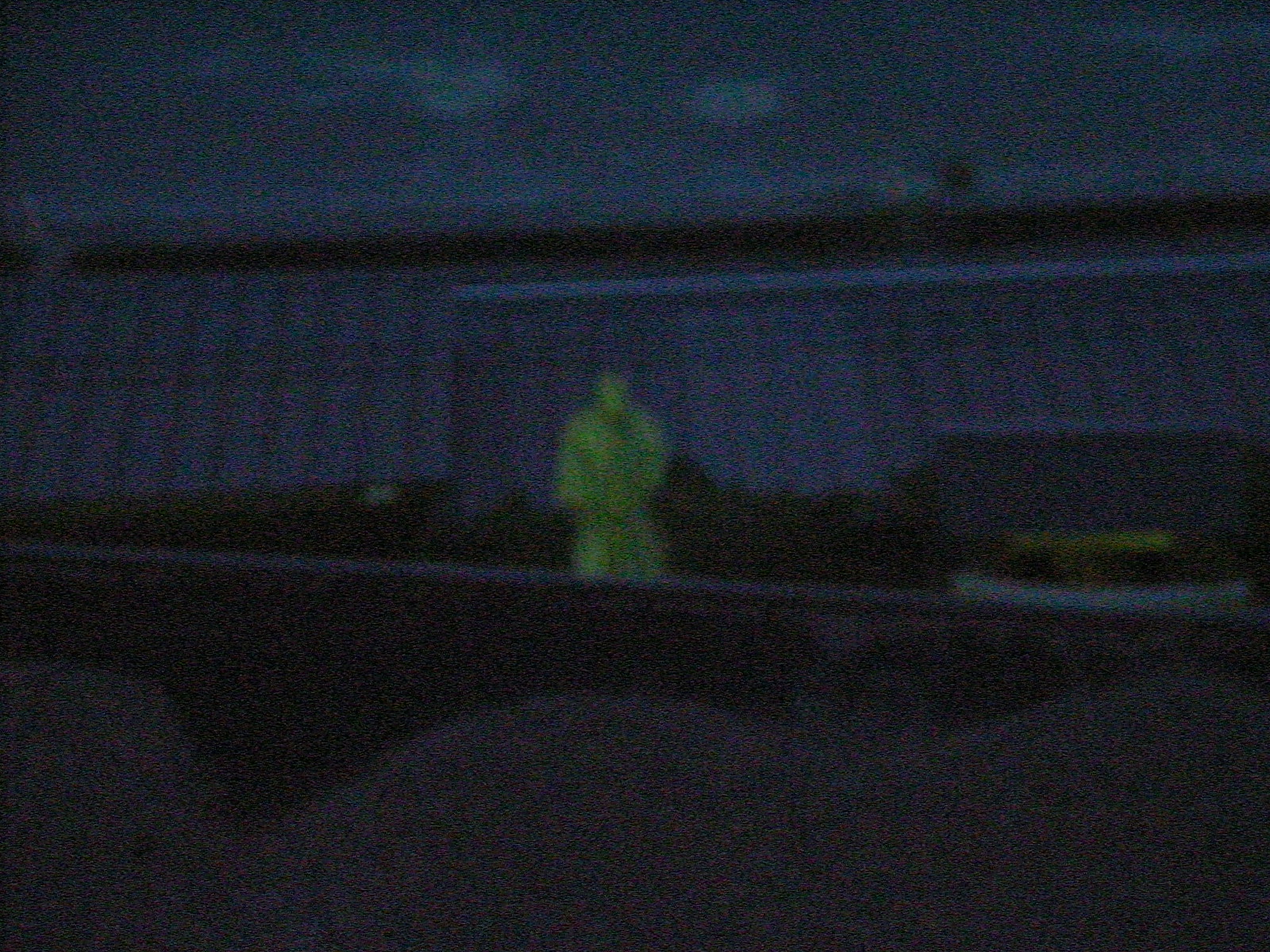The image depicts a scene that appears to be from a video game or computer game, taken at night. Central to the image is a character resembling a green army man, potentially dressed in a yellow-green trench coat with a hood. The background features what looks like a rooftop amidst a dark, blurry, and grainy environment, indicating poor image quality. The sky above is dark, speckled with white patches, possibly clouds. Below the dark rooftop edge, there is a lined structure with a silver rod, and beneath this, various rectangular sections, which may be part of a building or train cars. At the forefront are dark wavy mounds, adding to the obscured, night-time setting of the scene.